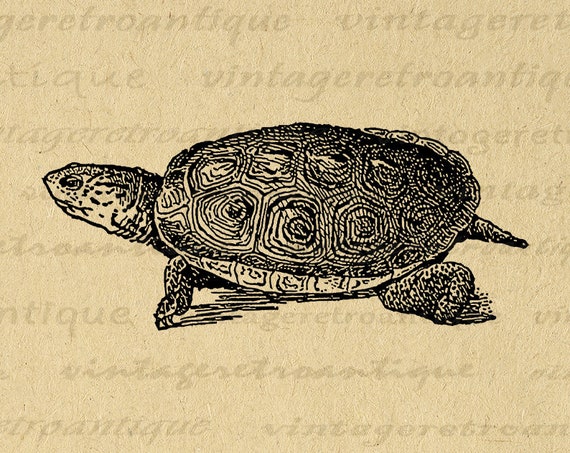This image is an illustration of a turtle rendered in a stylized manner with bold, dark lines that define its overall shape and features. The turtle has a sturdy, domed shell adorned with a pattern of swirls and ten distinct circles that give it a textured and intricate appearance. The turtle's head, featuring a pointed snout and open eye, is slightly extended but not fully out of its shell. Its front and back legs are splayed out to the sides, and each foot has clearly drawn, stubby toes with little claws. A cone-shaped tail is visible at the back.

The background of the image resembles sepia-toned or brown textured paper, creating a rustic or vintage ambiance. This vintage feel is enhanced by the presence of a repetitive watermark saying "Vintage Retro Antique" in various fonts, stretched horizontally across the image. Additionally, black lines at the bottom of the turtle suggest movement or indicate its shadow. The overall effect is simple yet charming, capturing the essence of the turtle with a nostalgic, antique quality.